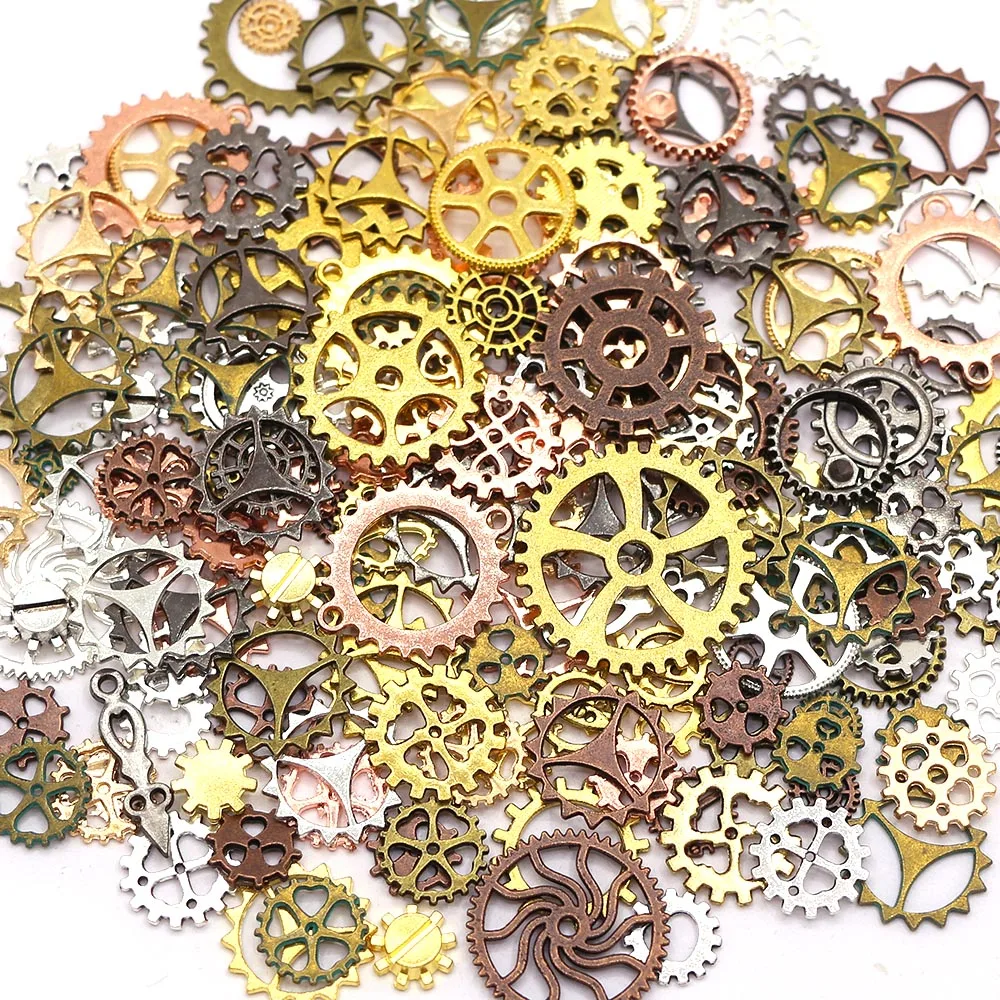This detailed photograph, oriented in portrait mode, vividly displays a large pile of variously colored and intricately designed gears and sprockets set against a light gray background. Amidst the pile, we find a diverse palette including bright gold, dark bronze, copper, silver, dark black, and shades of peach and olive, evoking a distinct steampunk aesthetic. The gears vary in size and shape, and their configurations range from simple circular forms to more complex designs with spokes and intricate inner patterns. Notably, the gears feature circular outer rings with teeth-like notches. A large brown gear with a spiral inner hole is prominently positioned at the bottom center, while directly above it, a smaller bronze gear with a triangular center catches the eye. Above these, a significant gold gear with five spokes around its center hole stands out. The gears overlap, creating a dense and layered composition. Interestingly, near the bottom left, slightly upward, lies a unique dagger-shaped object, subtly different from the gears. The photograph’s realistic representation captures the detailed textures and metallic sheen of each gear, making it a fascinating visual for steampunk enthusiasts, cosplayers, and admirers of detailed mechanical art.